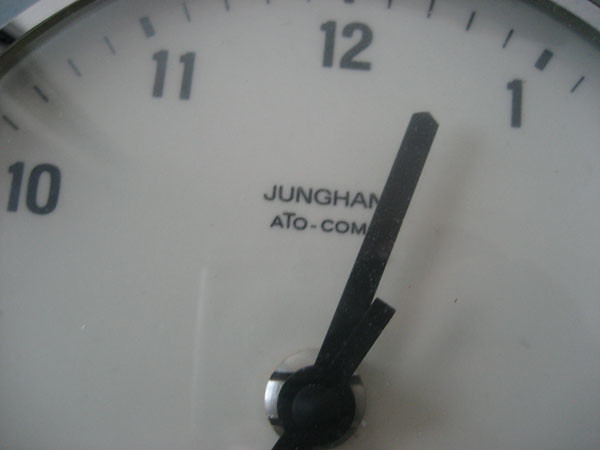Zoomed-in on a square-shaped clock, this image, despite its lower resolution, clearly displays unique details. The clock face features black numerals arranged in a counterclockwise manner, starting from the left with 10, 11, 12, and then 1. Black line markers designate each hour. Centered on the face, the text "JUNGHANS" is prominently displayed, spelled out as J-U-N-G-H-A-N-S, with "ATO-COM" situated below it, both in black. The clock hands, also in black, are visible and contribute to the overall monochromatic theme.